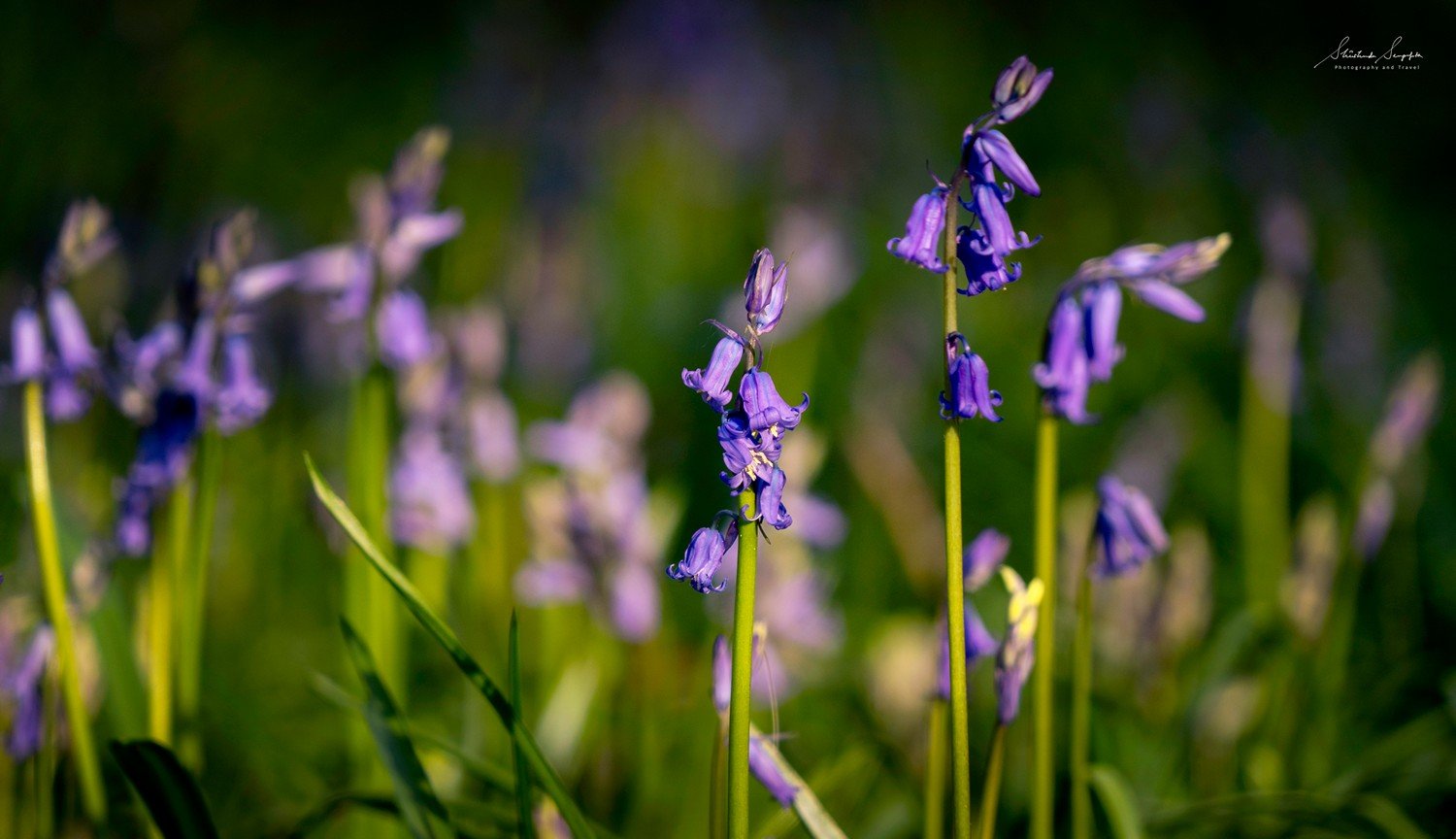This photograph captures a lush field of vibrant purple foxglove flowers, predominantly blurred to create a dreamy backdrop with striking focal points. The bell-shaped flowers, growing in healthy clusters, bloom from several sections of tall, light green stems reaching three to four feet in height. The stems emerge straight up from the ground, adorned with these graceful blooms. A few blades of grass are also in focus, adding texture to the scene. While most of the image is a beautiful wash of green and purple, two prominent flower stalks stand sharply in focus at the forefront, illustrating the intricate details of the bright purple petals and green stalks. An indecipherable name appears subtly in the top right corner, giving the image a hint of mystery amidst its natural beauty.